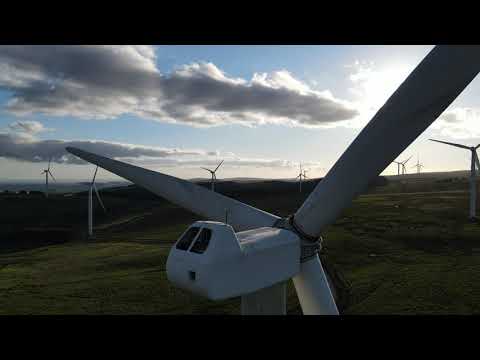This aerial photo captures the expansive beauty of a wind turbine farm during the daytime, likely around sunset, as indicated by the shadows cast on the ground. The main focus is a prominent wind turbine, viewed from the top, facing away from the camera. This central turbine showcases its three large white blades, typical of such eco-friendly designs. Surrounding this focal point, strategically placed along the green hillside, are six to ten additional wind turbines, all similarly equipped with three blades. The farm spreads across a landscape dotted with some trees and covered in green grass. The sun is partly obscured by one of the blades, contributing to the semi-cloudy ambiance of the scene. This innovative renewable energy setup clearly blends into the natural surroundings, emphasizing both technological progress and environmental harmony.